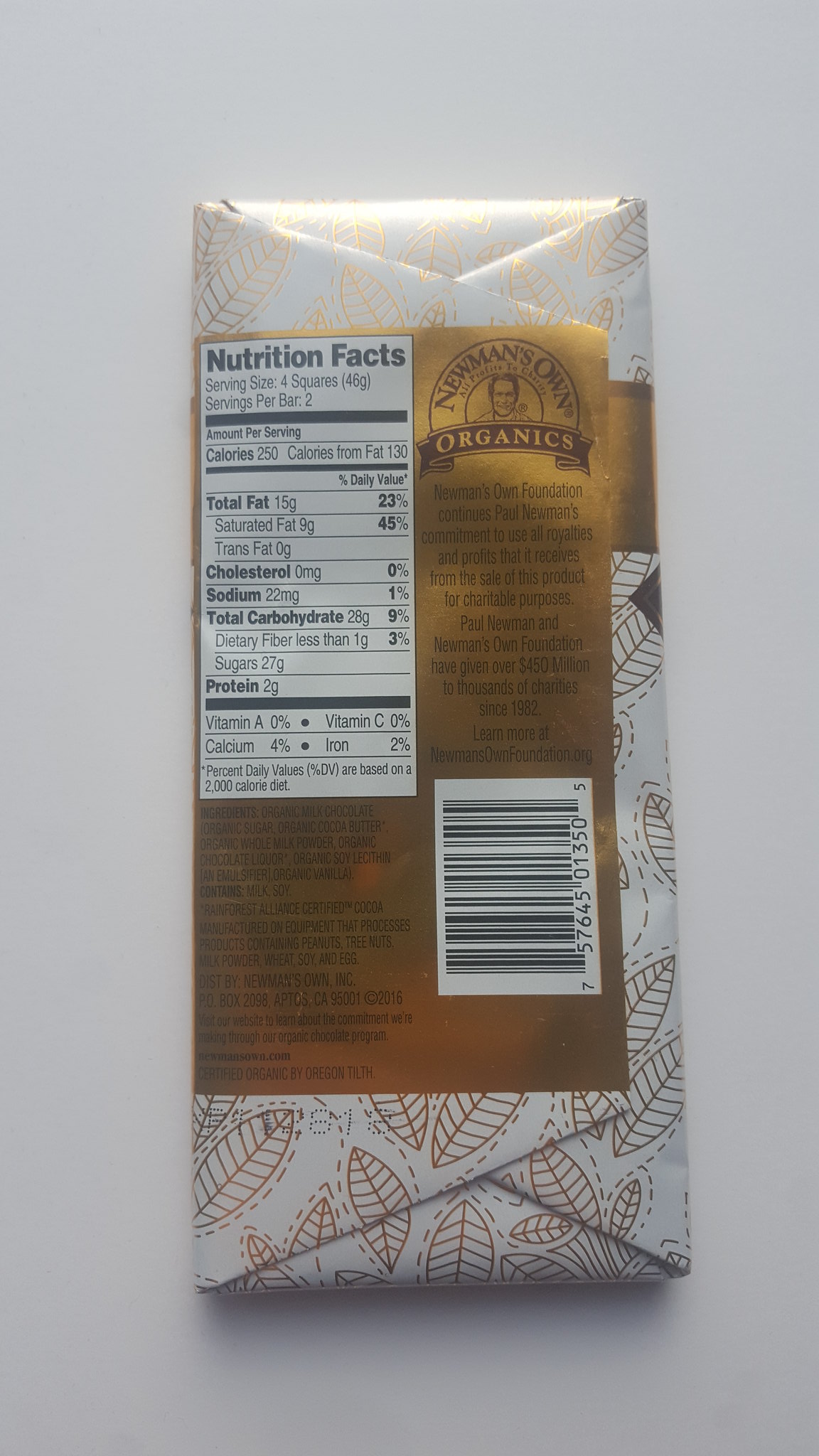The image is a close-up, color photograph of the back of a food product, which appears to be an organic chocolate bar. The package is primarily white with an intricate design of golden leaves scattered across it. Central to the wrapper, a gold section features text and a circular logo of Paul Newman. The logo and text are in brown, highlighting the Newman's Own Organics brand. Detailed nutritional facts are prominently displayed in a black and white rectangle, specifying that the serving size is four squares (46 grams), with two servings per bar. Nutritional information includes 250 calories per serving, 15 grams of total fat, 9 grams of saturated fat, 22 milligrams of sodium, 28 grams of carbohydrates, 27 grams of sugar, and 2 grams of protein. The package also emphasizes that all profits from the product are donated to charity through Newman's Own Foundation, which has contributed over $450 million since 1982. A white barcode is positioned below the text, adding to the structured back panel of the wrapper.